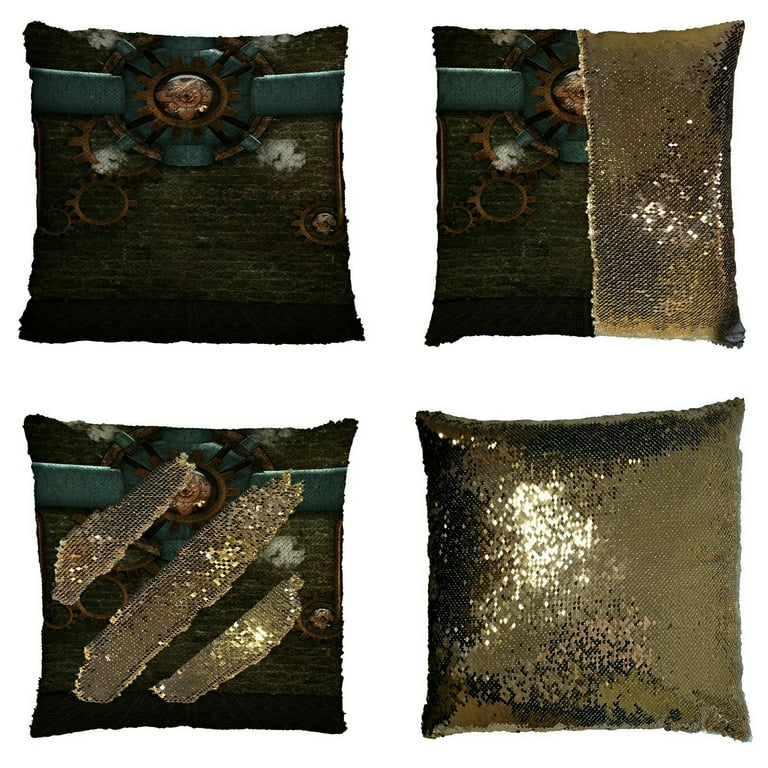The image showcases four decorative pillows arranged in a grid against a white background, each occupying one quadrant. These pillows are adorned with reversible gold sequins, which shimmer and create a dynamic visual effect. The sequence reveals a unique printed design on the non-sequin side, depicting a dark brown brick wall texture with some rusted metal gears and a dark teal geometric shape at the top. 

In the top left quadrant, the pillow is fully displaying this intricate design. The top right pillow illustrates the transition, displaying half of the brick wall image on the left while the right half is covered in glittering gold sequins. The bottom left pillow adds another variation, featuring three diagonal lines where the sequins have been flipped to reveal gold, contrasting against the printed image. Finally, the bottom right pillow is entirely covered in shimmering gold sequins, hiding the intricate design beneath and showcasing the versatility and luxurious aesthetic of the pillows.